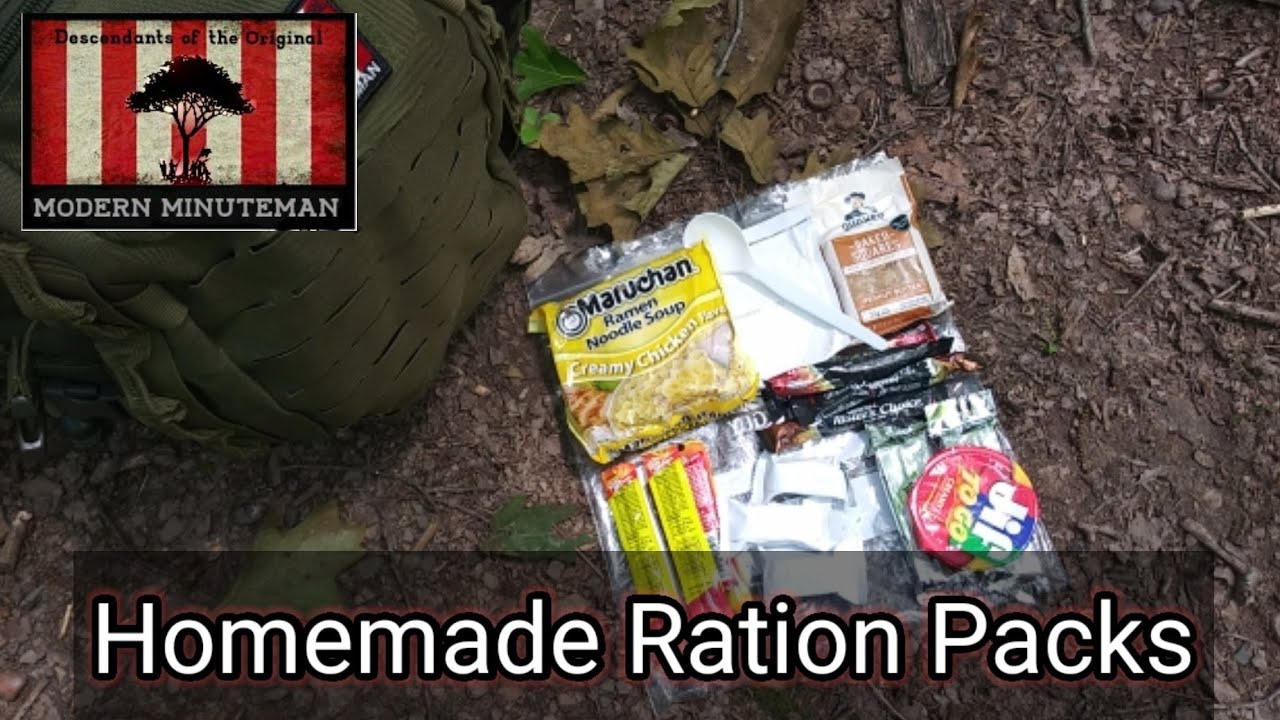The photograph features a natural outdoor setting with a dirt background scattered with leaves, twigs, and some green foliage. Prominently displayed on the ground is a green backpack positioned in the left-hand corner. In the center lies a plastic bag that appears to be a sample homemade ration pack. This pack includes several items: a yellow package of Maruchan Ramen Noodle Soup in creamy chicken flavor, a plastic white spoon, a small container of Jif To-Go peanut butter, and packets of oatmeal and beef jerky or Slim Jims. At the bottom of the image, white text reads "homemade ration packs". In the upper left-hand corner, there is a rectangular graphic featuring red and white stripes with a black tree. Above the tree, black text reads "descendants of the original", and below it, in white text, "modern minute men".